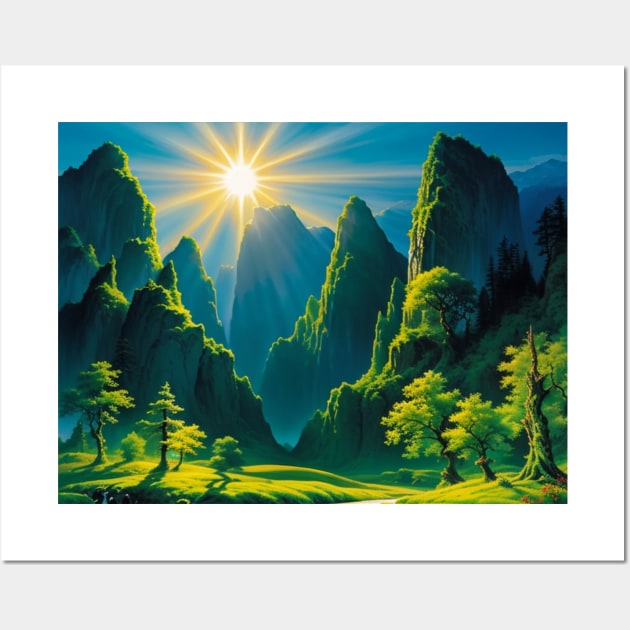This product photo showcases a beautifully illustrated print centered on a white wall. The illustration features a picturesque scene dominated by green and blue hues, depicting a vibrant forest nestled among layered mountain ranges. The mountains, covered in lush vegetation, extend into the distance, their deeper blue shades contrasting with the rich greenery in the foreground. The sun, depicted with a bright yellow center and radiating rays, illuminates the scene, casting a warm, yellowish glow that highlights the trees and grass below. The sun's rays are spread individually, creating an intricate play of highlights and shadows throughout the landscape. The entire illustration is encased in a white border, adding to its overall charm and festive, vibrant ambiance. The style leans towards a cartoonish or hand-drawn aesthetic, emphasizing a delightful and detailed depiction of nature.